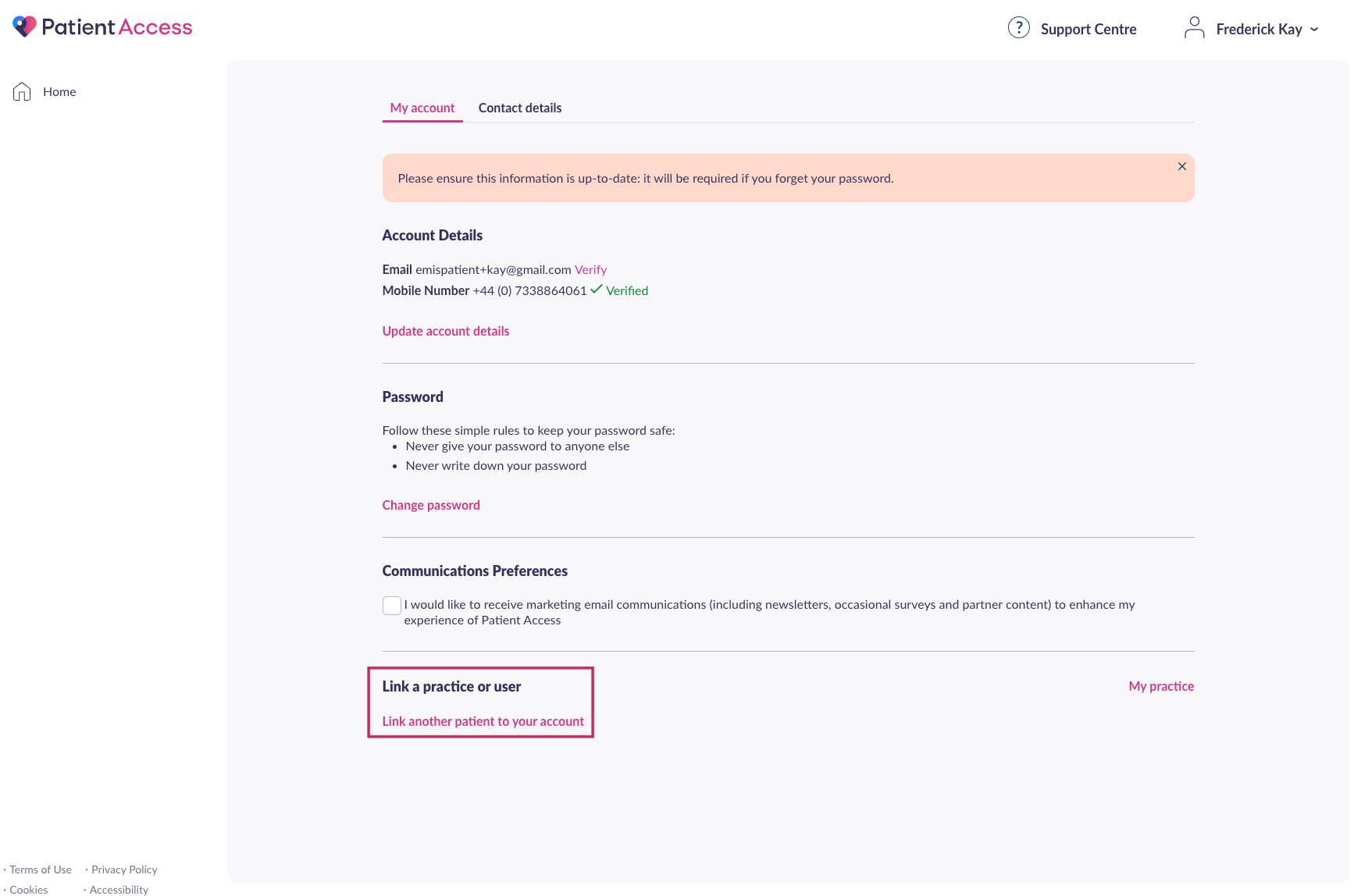The image presents a web interface for a "Patient Access" section, set against a grayish background. At the top, the term "Patient Access" is displayed, with "Patient" in navy blue and "Access" in pink. A heart icon is positioned in front of the text, divided into sections: one-quarter navy blue, one-quarter teal, and half pink.

Moving to the next section on the interface, there is a "Support Center" area mentioning a user, "Frederick K." Below this, a salmon-colored box contains the instruction: "Please ensure this information is up-to-date. It will be required if you forget your password."

Further down, there are sections for account details and security. The "Account Details" section lists email and mobile number fields. The email is followed by a pink "Verify" button, and the mobile number is marked with a green check indicating it’s verified. There is also a pink "Update Account Details" button.

The "Password" section advises on creating a secure password, including tips like never sharing or writing it down. A pink "Change Your Password" button is provided. 

Next, the "Communications Preferences" section allows users to opt-in to receive marketing emails, newsletters, surveys, and partner content by checking a box, which is currently unchecked. 

The "Link a Practice or User" section is highlighted in pink, offering options to link another patient to the account. Lastly, on the right side, there is a "My Practice" section labeled in pink.